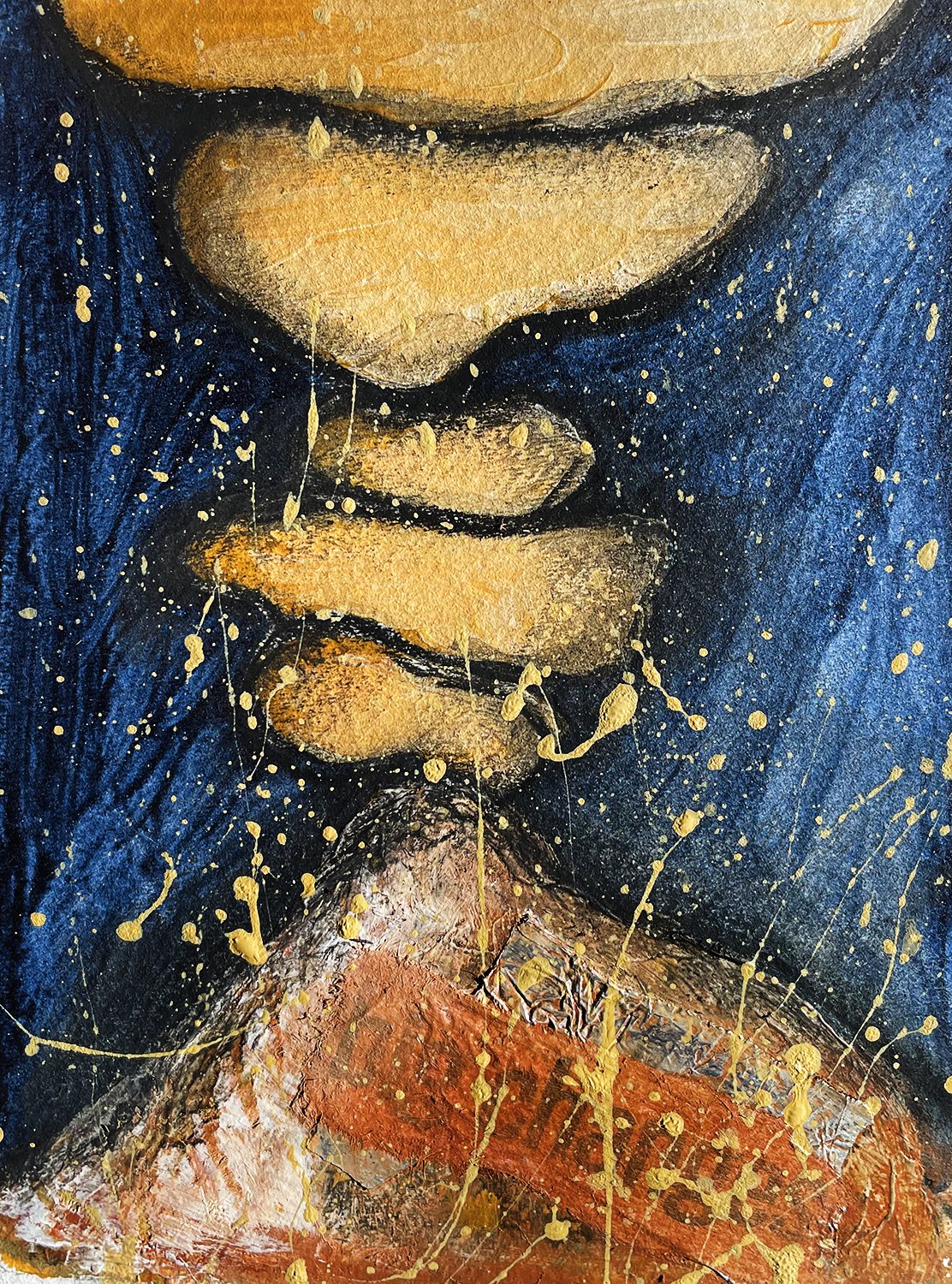This is a detailed painting, presented in a portrait orientation that is taller than it is wide. The artwork features an abstract representation that evokes various interpretations. At the bottom, there is a maroon and brown rock-like object with a pointed end. This base structure supports a series of lighter, yellow-colored rocks stacked on top of each other, alternating in size from smaller to larger and extending off the top of the canvas. These rocks are bordered in black and have a textured appearance, with each brush stroke distinctly visible. One of the rocks even features a red sticker that says "big change." Surrounding the main objects, there's a dynamic blue sky in the background, filled with streaks of different shades of blue. Additionally, the entire canvas is sporadically adorned with gold paint splatters, which are denser towards the middle and bottom portions of the painting, becoming sparser as they approach the top. This combination of elements and textures gives the painting a sense of both chaos and balance, drawing the viewer into its layered depths.